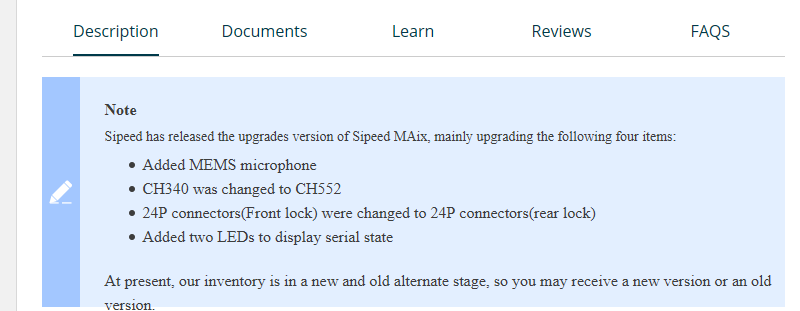A rectangular image with the longer sides extending horizontally is described. A gray vertical border runs along the left side of the image. At the top right, a header featuring the words "Description," "Documents," "Learn," "Reviews," and "FAQs" is displayed, with "Description" being underlined. A thin gray line separates this header from the content below.

Continuing down, there is a prominent blue box with a darker blue vertical border on the left side. Within this border is a white pencil icon. The main content in the section reads as follows in black text:

"Note: Sipede has released the upgraded version of Sipede MAIX, with the following four improvements:
- Added MEMS microphone
- CH340 was changed to CH552
- 24P connectors (front lock) were changed to 24P connectors (rear lock)
- Added two LEDs to display serial state

At present, our inventory consists of both new and old versions alternating, so you may receive either version."

This descriptive caption aims to convey all the crucial elements present in the image accurately and in detail.